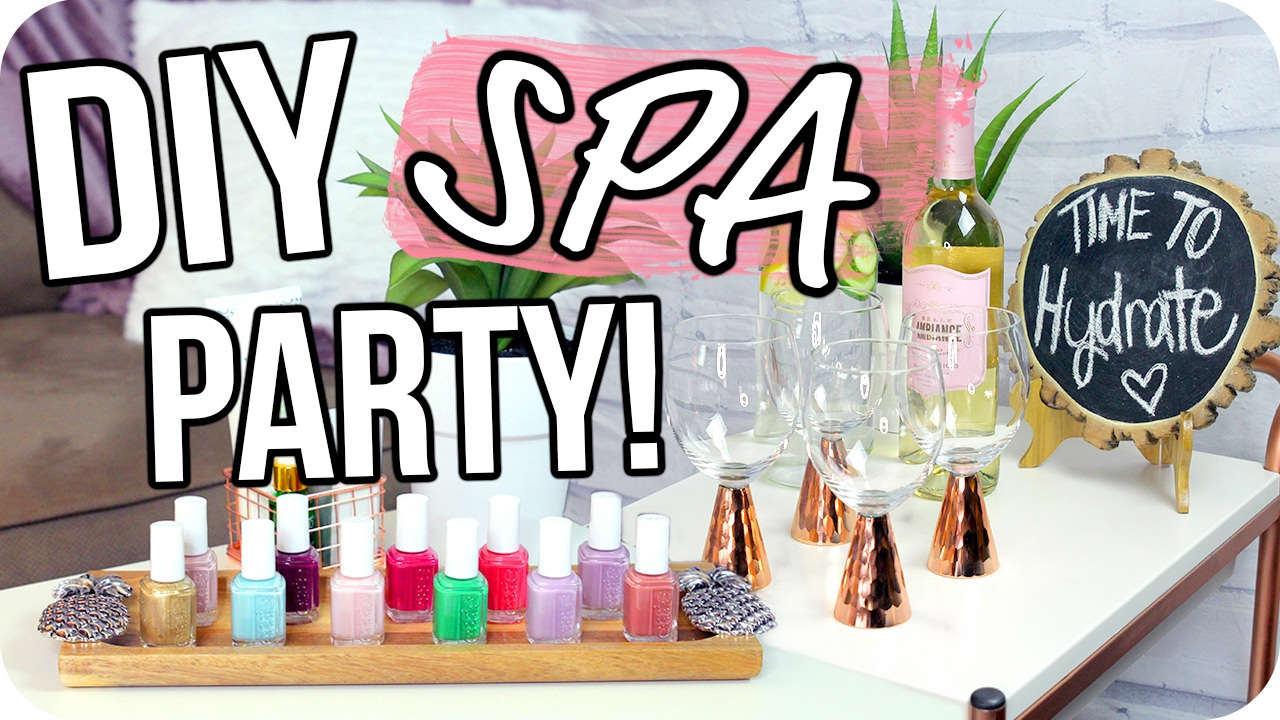The horizontally aligned rectangular image features a vibrant advertisement for a DIY Spa Party, with large, all-caps white block letters outlined in black, prominently placed in the upper left corner and extending to the middle, reading "DIY SPA PARTY!". An exclamation mark punctuates the excitement. The background showcases a light gray brick wall within an indoor room setting. 

Central to the image is a white table with brown wooden legs, adorned with a variety of colorful items. On the left side of the table sits a rectangular wooden tray filled with numerous bottles of nail polish, each sporting white lids. The nail polishes come in a spectrum of colors, including gold, baby blue, soft pink, bright green, and lavender, adding to the scene's vibrancy. 

To the right of the nail polishes are four wine glasses with elegant conical gold bottoms and clear glass tops, positioned beside a bottle that appears to be champagne, identifiable by its pink label and top. At the table's corner stands a small circular chalkboard displaying the message "time to hydrate" written in white chalk, accented with a heart symbol.

In the background, a green aloe plant adds a touch of nature to the otherwise festive and luxurious setting. With its myriad of colors—pink, black, gold, purple, red, green, white, blue, and yellow—the image beautifully captures the essence of a celebratory and relaxing spa party.